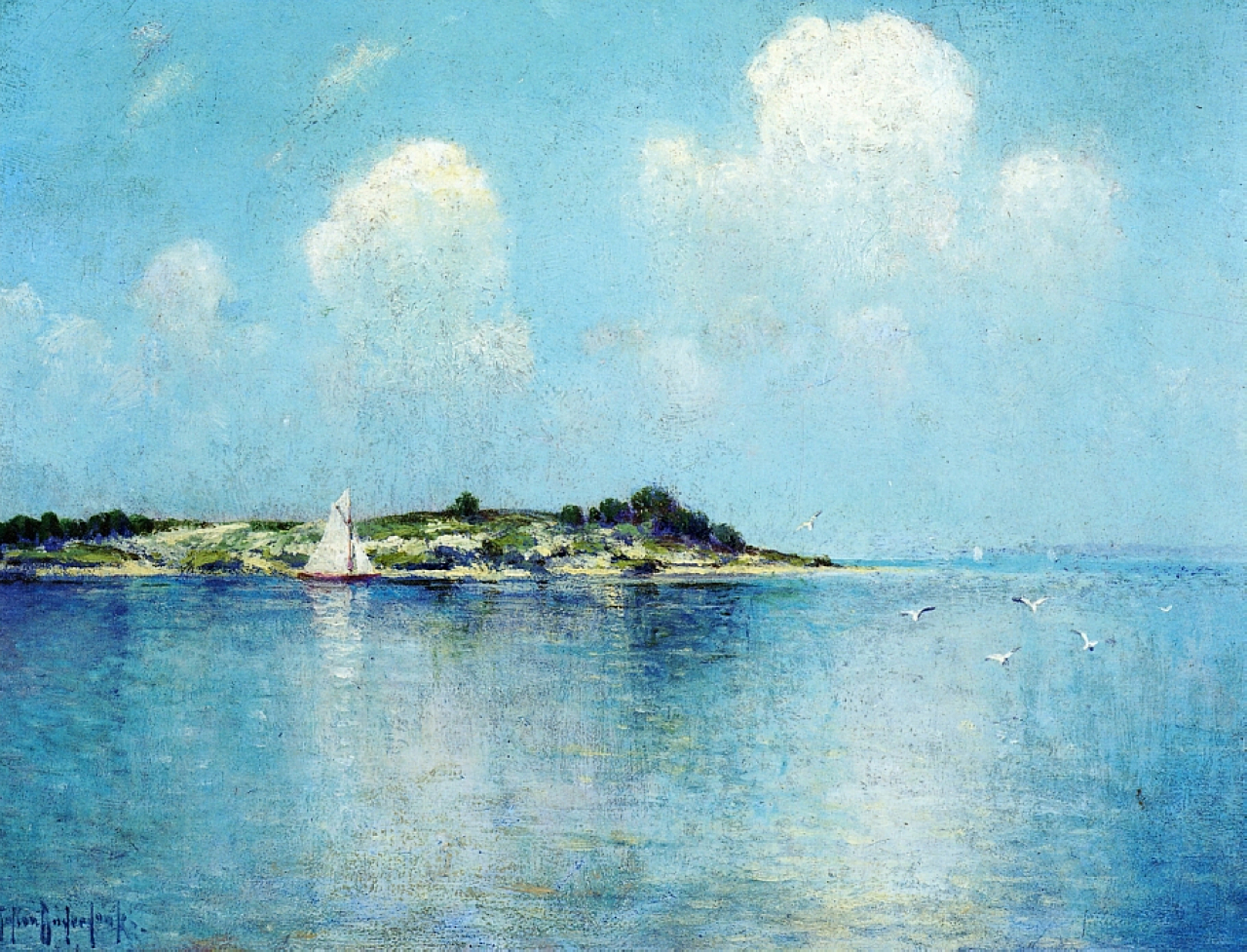The painting showcases a serene maritime scene under a clear blue sky dotted with soft, white clouds. The top half of the artwork is dominated by this vibrant sky, where the clouds seamlessly fade into the horizon. Below, there is a green peninsula extending into a vast body of blue water, the island's reflection mirroring in the calm waves. On the left side of the image, close to the shoreline, a distinctive red sailboat with white triangular sails stands out. On the right, four seagulls with white and dark-tipped wings hover above the water. The sea stretches beyond, with faint land possibly in the distant background, contributing to the artwork's expansive feel. The painting's texture is visible, notably in the brushstrokes that bring depth to the elements, enhancing the lifelike quality of the scene. A signature resides in the bottom left corner, adding a personal touch to this peaceful coastal vignette.